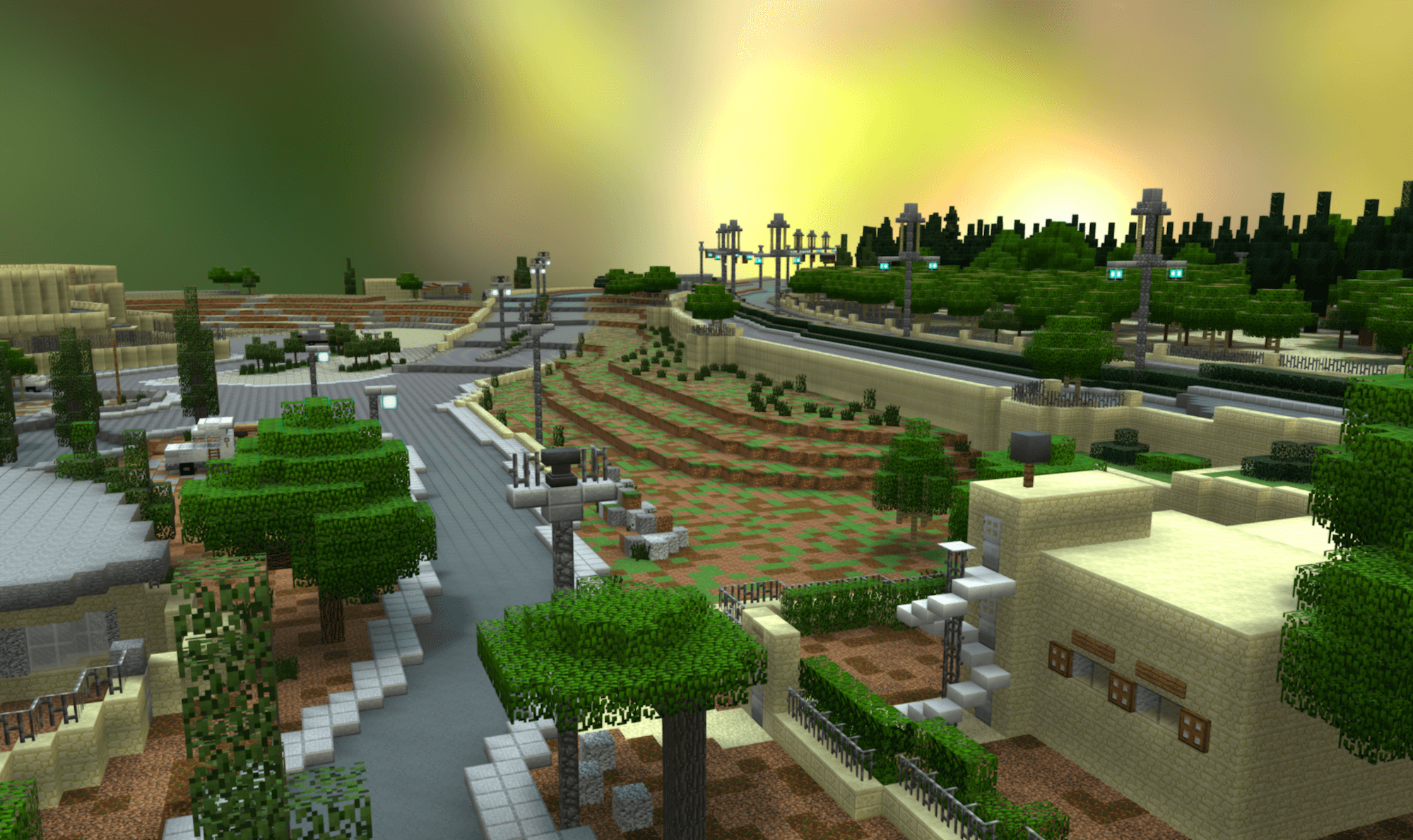In this image, we see a detailed and expansive virtual cityscape, likely created in a blocky, pixelated style reminiscent of Minecraft or similar video games. The city is characterized by its geometric, Lego-like appearance with no humans in sight. Prominent features include a yellow stone building in the lower right corner, which has a white spiral staircase on the outside and a yellow stone fence topped with metal. The scene is adorned with various blocky, textured trees and bushes, as well as numerous gray and brick-like pathways, walkways, and staircases that traverse different levels.

A noticeable gray road, lined with white stones, runs along the left-hand side and ascends a series of stairs. On the far right, there is a highway or possibly a railroad line, flanked by many street lamps. The area is rich with landscaping—hedges and low, square buildings are scattered about, creating a terraced or leveled appearance. In the blurred, glowing background, which might be illustrative of a wildlife photo or simply an out-of-focus backdrop, dark shapes suggest either distant trees or structures. The sky displays a blend of colors—green, yellow, white, and brown—adding to the fantastical, dreamy atmosphere of the scene.